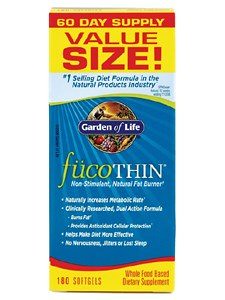This image features a prominently displayed box of dietary supplements branded "Garden of Life." The product packaging, characterized by vibrant colors such as red, yellow, blue, white, and a bronzy-orange, claims to offer a "60-day supply" in a "value size." It highlights that it is the "number one selling diet formula in the natural products industry" and identifies the product as "FucoThin," a "non-stimulant natural fat burner." While some of the text is unclear, essential information such as "180 soft gels" and "whole food based dietary supplement" is visible. The "Garden of Life" logo, enriched with detailed imagery of fruits—grapes, an apple, and possibly a plum—alongside a carrot, sits above a globe-like background, reinforcing the brand’s natural and holistic imagery. The overall presentation of the box is clean and straightforward, front and center against an unobtrusive background, likely intended for advertising purposes.